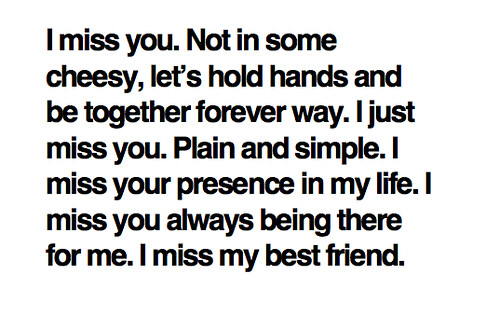The image consists of plain black text on a white background, written in a bold, sans-serif font, likely Arial. The text delivers a heartfelt message, stating: "I miss you. Not in some cheesy, let's hold hands and be together forever way. I just miss you, plain and simple. I miss your presence in my life. I miss you always being there for me. I miss my best friend." This straightforward and emotive note, composed of roughly 40 words and spanning across several sentences, encapsulates a deep sense of longing and friendship. There's no additional imagery or design elements; the focus remains solely on the powerful, English-phased message expressed in black bold font against the stark white backdrop. This sentiment can be fittingly shared on various mediums, such as a card, social media, or even as a decorative art piece.